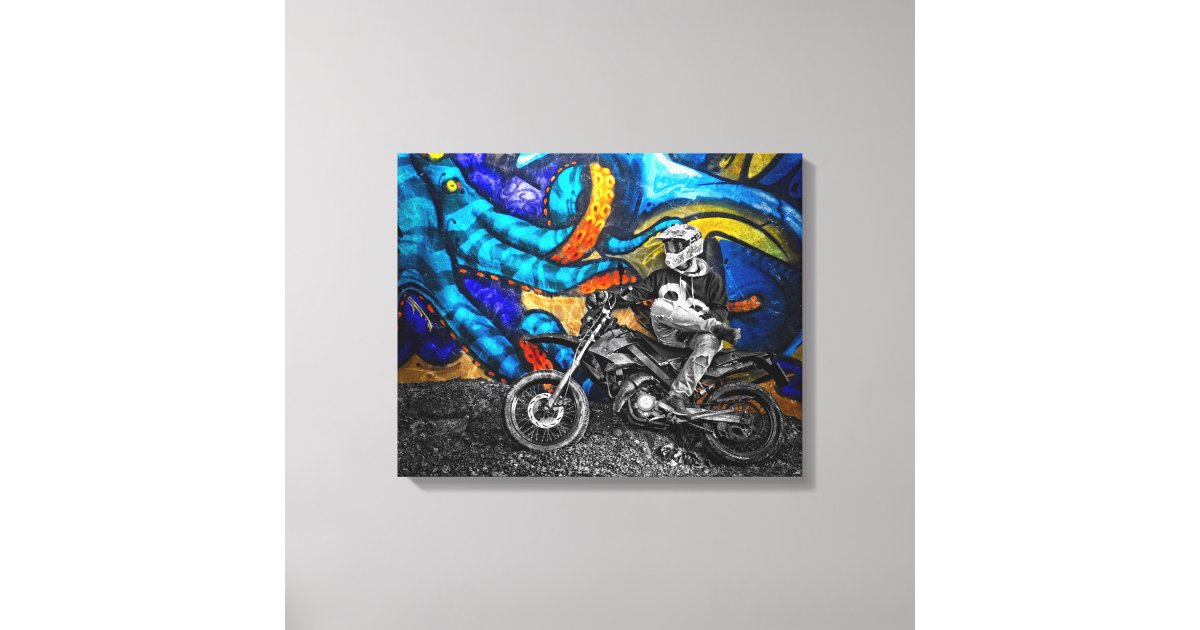This image showcases a striking piece of artwork hanging on a gray wall adorned with vibrant street art in a multitude of colors including whites, greens, purples, yellows, blues, and reds. Against this colorful backdrop, a man sits on a gray, black, and white motorcycle. He is positioned with his right leg casually crossed over his left knee and his left foot propped on the motorcycle's parts. Dressed in a black jacket and wearing a helmet, the man is situated on a gravel patch, adding depth and texture to the scene. The photograph captures the juxtaposition of the vivid mural and the monochromatic motorcycle and rider, creating a visually engaging composition.